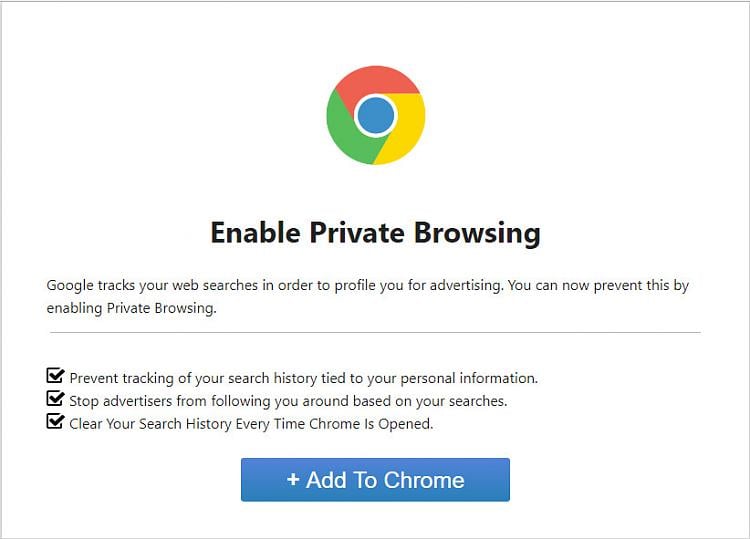Screenshot of a computer screen displaying a Google Chrome settings page:

At the top, a prominent Google Chrome icon is featured. The icon displays a teal blue circle in the center, encased by a thin white circle, and encircled by segments of red, yellow, and green forming a larger outer circle. Below the icon, bold black text instructs, "Enable private browsing." Smaller print beneath this explains, "Google tracks your web searches in order to profile you for advertising. You can now prevent this by enabling private browsing."

A faint gray horizontal line separates this section from the one below. This lower section contains three vertically-aligned checkboxes, all marked with black check marks. The checkboxes are labeled with the following statements:

1. "Prevent tracking of your search history tied to your personal information."
2. "Stop advertisers from following you around based on your searches."
3. "Clear your search history every time Chrome is opened."

At the bottom of the screen, a blue rectangle button displays the text "Add to Chrome" in white print.